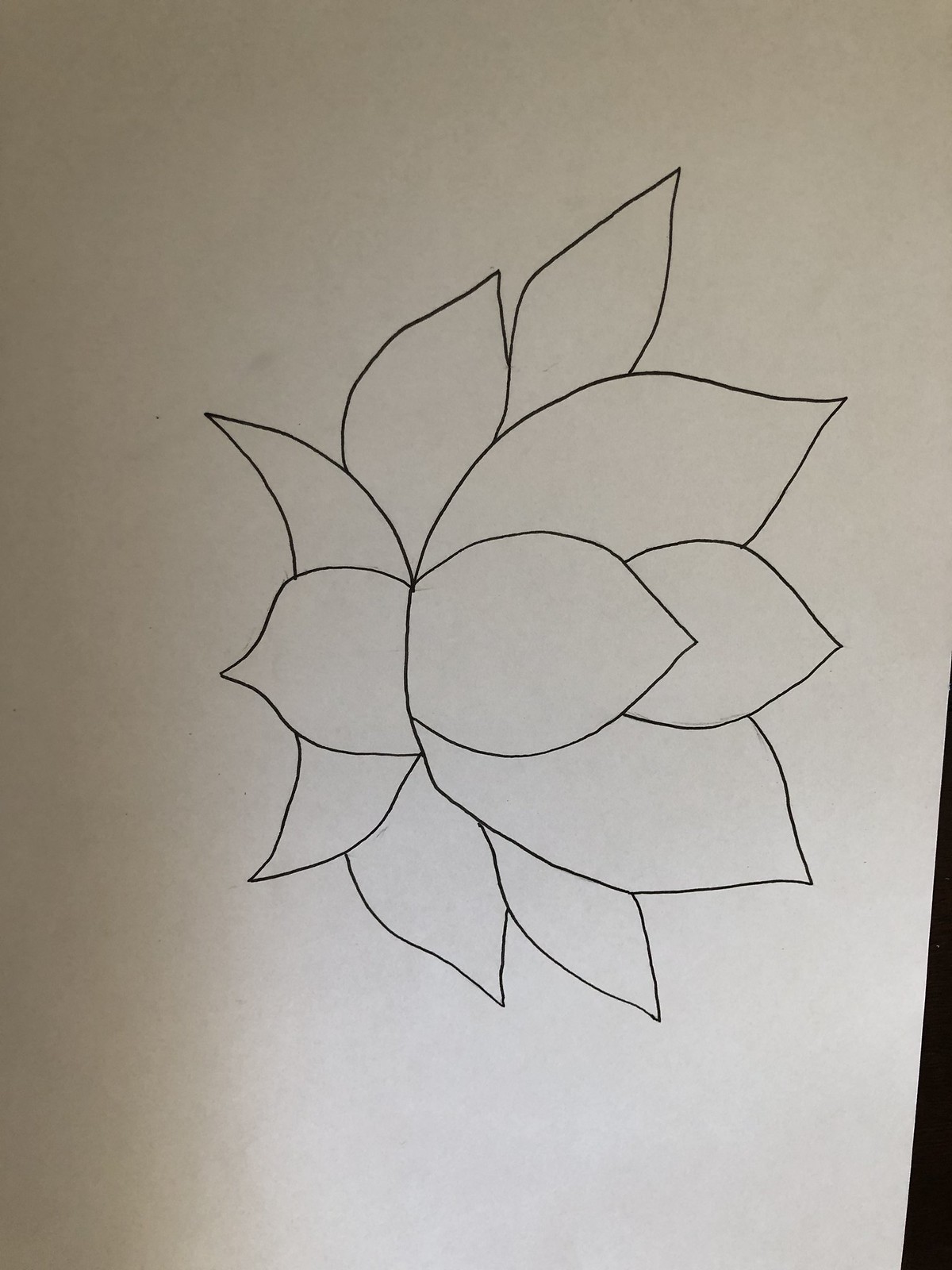This is a photograph of a pencil sketch on a piece of white printer paper, which appears slightly transparent with a shadow down the left side. The paper is positioned vertically, although it should ideally be horizontal, and it rests on a dark brown table visible in the bottom-right corner. The table is so dark it almost looks black due to the paper's angle. The sketch depicts the top part of a flower bud in black pen, featuring a detailed arrangement of petals. There are a total of eleven petals radiating from a central point, with eight larger petals forming the outer layer and being notably centered from the left to the right. In the middle, two teardrop-shaped petals overlap, each pointed at the ends, enhancing the depth of the drawing. The flower is depicted from a side view, with the top of the blossom oriented towards the right side of the page. The photograph is not well-lit, adding a certain depth and shadow to the overall presentation.